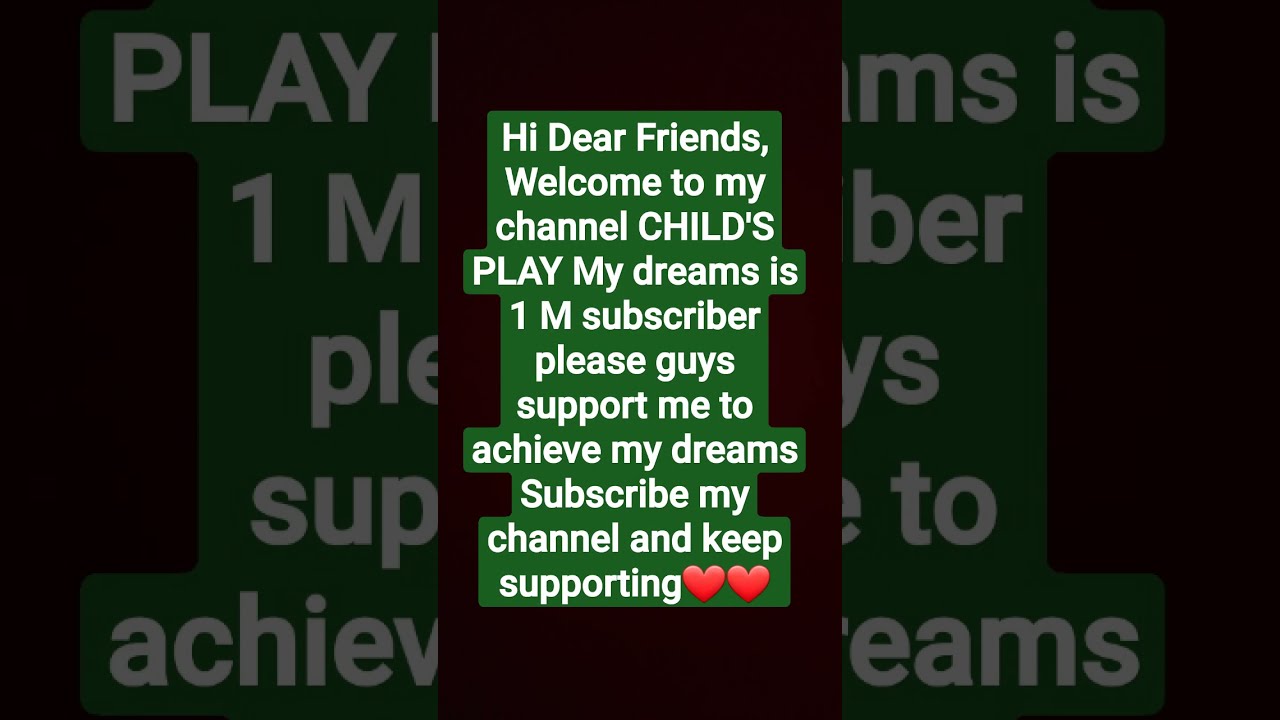The image displays a centered block of white text set against a completely black background, with portions of the screen showing partially obscured text on both sides. The main text reads: "Hi, dear friends. Welcome to my channel, Child's Play." The channel name "Child's Play" is in all caps. The message continues, "My dream is 1 million subscribers. Please, guys, support me to achieve my dream. Subscribe to my channel and keep supporting," and ends with two red hearts. This text is highlighted with a green outline, giving it prominence. The text capitalizes "Hi," "Welcome," "Dear friends," "My," the "M" in "1M," and "Subscribe." The image appears to be a screenshot taken from a mobile app such as TikTok or Instagram, with minor portions of the text visible along the edges due to the zoomed-in effect of the screenshot.